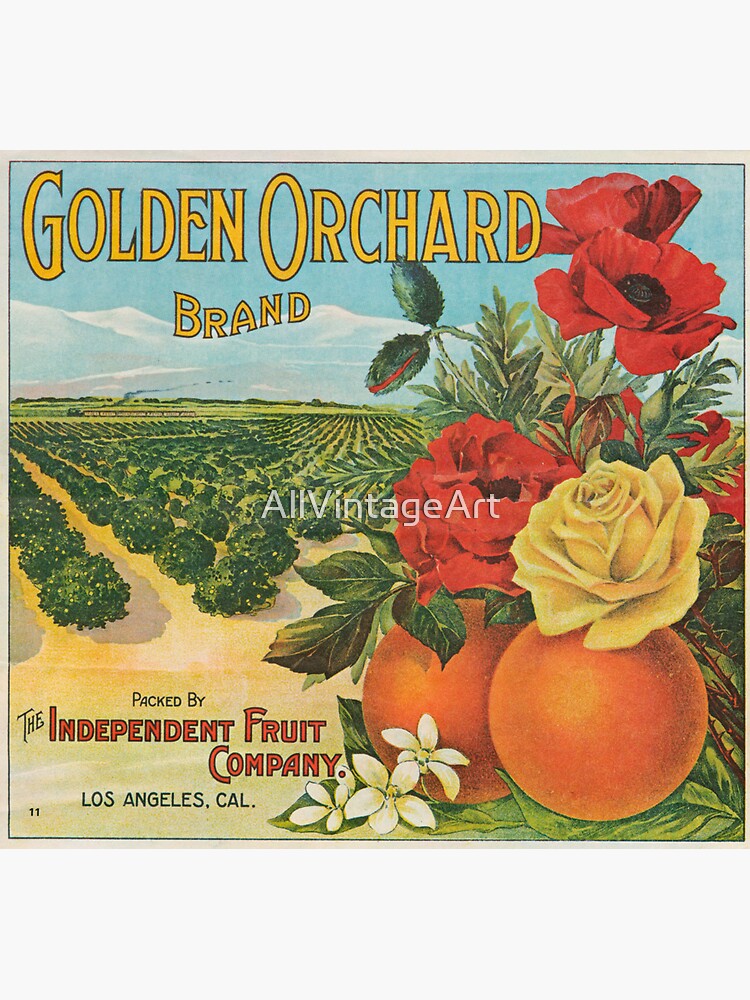The image is an old, square-shaped cover titled "Golden Orchard Brand," featuring vintage art with darker undertones characteristic of the period. Packed by the Independent Fruit Company in Los Angeles, California, the cover prominently displays a vivid scene in the foreground: two large oranges flanked by small white flowers, a yellow rose, a red rose, and possibly poppies amidst lush green leaves. Rising in the background are rows of trees and bushes, likely orange trees, extending as far as the eye can see. Above this pastoral setting, white mountains and a blue sky stretch across the horizon, adding depth to the vintage landscape. The number 11 is seen in the lower left corner, and a watermark states "All Vintage Art," further confirming its historic charm.